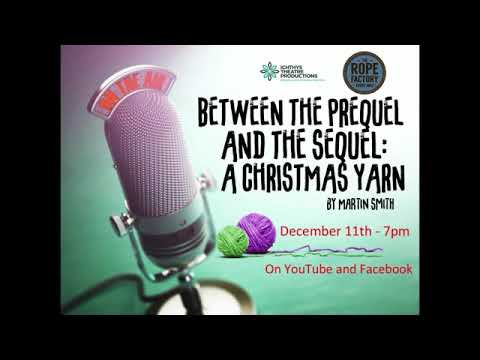This vibrant advertisement promotes the theatrical production "Between the Prequel and the Sequel: A Christmas Yarn" by Martin Smith, slated for a one-time broadcast on December 11th at 7 pm on YouTube and Facebook. The large uppercase black font highlights the title prominently in the center of the image. Above the title, there's a logo featuring "The Rope Factory" inside a blue circle with a black outline, and to its left, a small, possibly unreadable theater production logo. A striking visual on the left side features a metallic microphone with the words "On the Air" in red, creating an impression of a live broadcast. Beneath the title, the event's date and time are displayed in red script for clear visibility. Enhancing the festive spirit, there are colorful illustrations of two balls of yarn—a small green ball in front and a larger purple ball behind. The background features a light aqua gradient transitioning to a light purple gradient, adding a whimsical touch to the overall design.